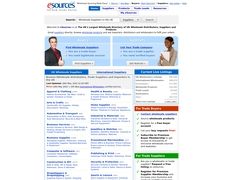The image depicts a website with an entirely white background. At the top center, the word "eSources" is prominently displayed, with "e" in a vibrant orange or red color and "sources" in blue. The text and images throughout the site are extremely small and heavily blurred, making specific details difficult to discern.

Directly below the "eSources" heading, there is additional text followed by a blue banner that appears clickable. Beneath this banner are four lines of unclear content. Further down, there's a search bar, flanked by more text written in black.

The page is divided into two blue panels: the left panel features an image of a man, and the right panel shows a woman. Below these panels, there is a section consisting of two columns within a square layout. This section contains blue text and is capped by different color banners — a blue banner at the top left and right, a red banner in the middle, and a green banner at the bottom. Each banner is accompanied by words and text beneath it. Under the red banner, there are five check marks aligned next to another set of text. Despite the detailed structure, all content remains blurred and unreadable.